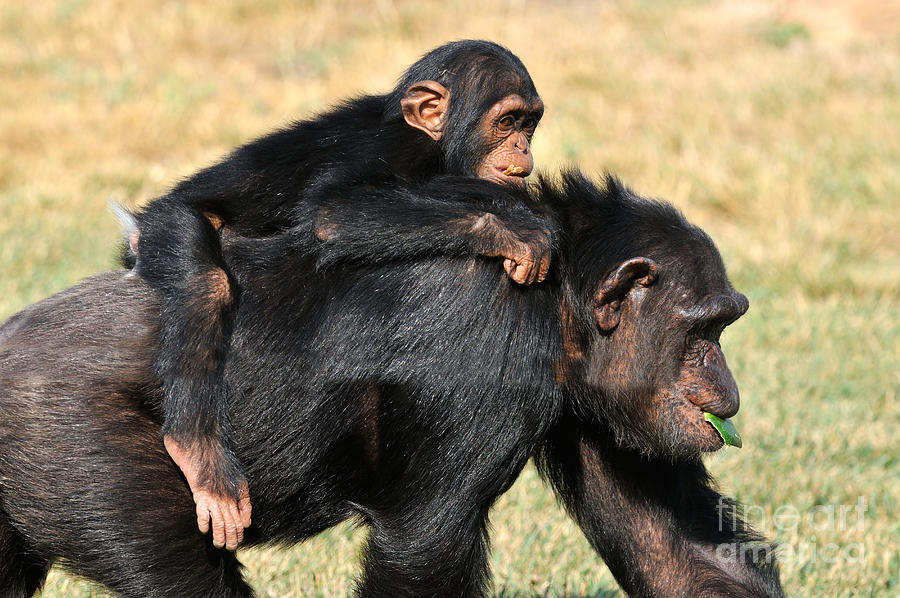In this captivating outdoor image, a mother gorilla is seen walking on all fours through a grassy area, with the foreground showing patches of green grass and the background consisting of blurred tan grass. Her fur is dark brown to black, and she holds a green leaf in her mouth, indicating she might be eating. Clinging to her back is a baby gorilla, also with dark fur. The baby has strikingly large ears and brown eyes, and it appears to have a bit of white fur at its tail end while its hands rest over the mother's shoulders. Both apes are seemingly on a journey, possibly searching for food or heading back to safety. This Fine Art America photo embodies the essence of these gorillas making their way through the wilderness.